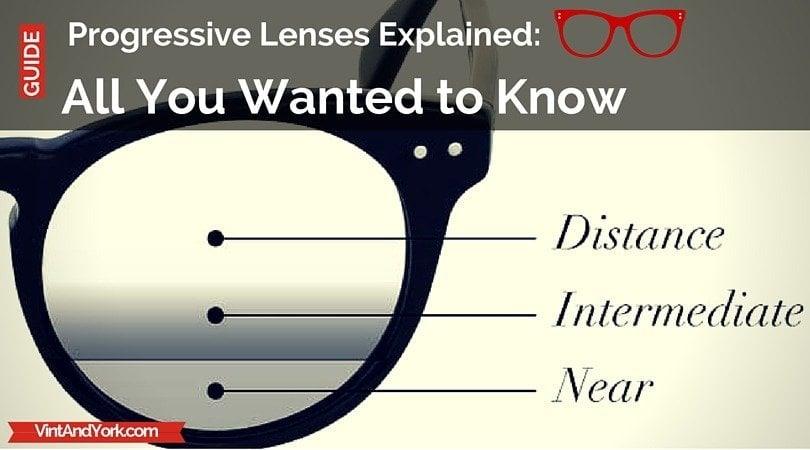The cover of this booklet on progressive lenses for eyeglasses features an informative and visually engaging design. The title, "Progressive Lenses Explained: All You Wanted to Know," is prominently displayed in white text against a dark gray background. A vertical red rectangle with white letters spells out "Guide," with the text running vertically from bottom to top. The booklet transitions into an ivory or beige color below the title, where a detailed black-framed eyeglass lens diagram is presented. The diagram illustrates the three vision zones on the lens: the top part labeled "Distance," the middle part "Intermediate," and the bottom part "Near." This diagram visually explains the functionality of progressive lenses. At the bottom left corner, within a small red banner, the manufacturer's website, VintandYork.com, is printed in white text. This grey, black, and ivory colored brochure combines both essential information and clear visual aids to serve as a comprehensive guide on progressive lenses.